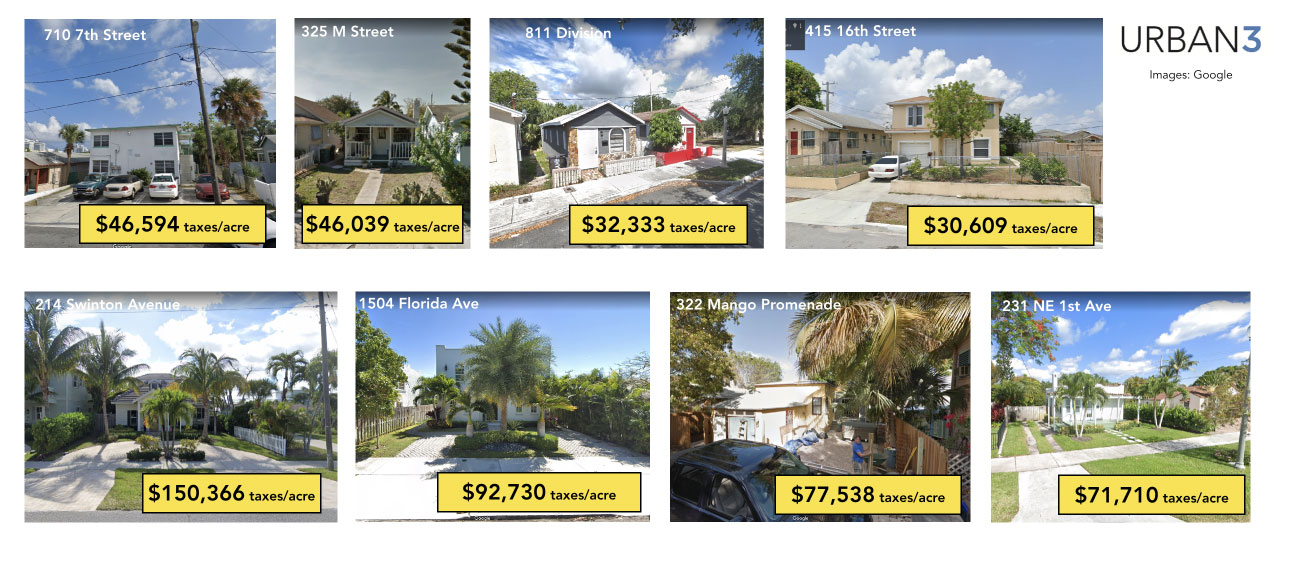The image features a white background with four distinct real estate listings at the top.

1. The first listing on the left showcases a white condo-like house with three cars parked in front—two white cars and one bluish-green. A telephone pole is visible towards the right side. The text "710 7th Street" is displayed at the top left. At the bottom right, there's a yellow label with a black border and bold black text reading "$46,594," and in smaller lettering, it says "taxes/acre."

2. The second image presents a more tropical setting, identifiable by the lush trees and a pathway flanked by lawns on both sides. A house, likely white or blue, with pillars is visible. The text "325 M Street" appears in bold white letters at the top left. At the bottom, there's a similar yellow label with bold black text reading "$46,039," and smaller text "taxes/acre."

3. The third image displays a street-side view from the right side of a gray house with a white door and a stone walkway. The text "811 Division" is shown in white at the upper left. A yellow label at the bottom right features bold black text reading "$32,333," and smaller text "taxes/acre."

4. The fourth image shows two beige houses, with the one on the left featuring red shutters. Text at the upper left reads "415 16th Street". A similar yellow label at the bottom right contains bold black text "$30,609," and smaller text "taxes/acre."

Overall, the detailed captions and consistent design elements such as the yellow labels with black borders and text provide quick reference points for discerning property details.